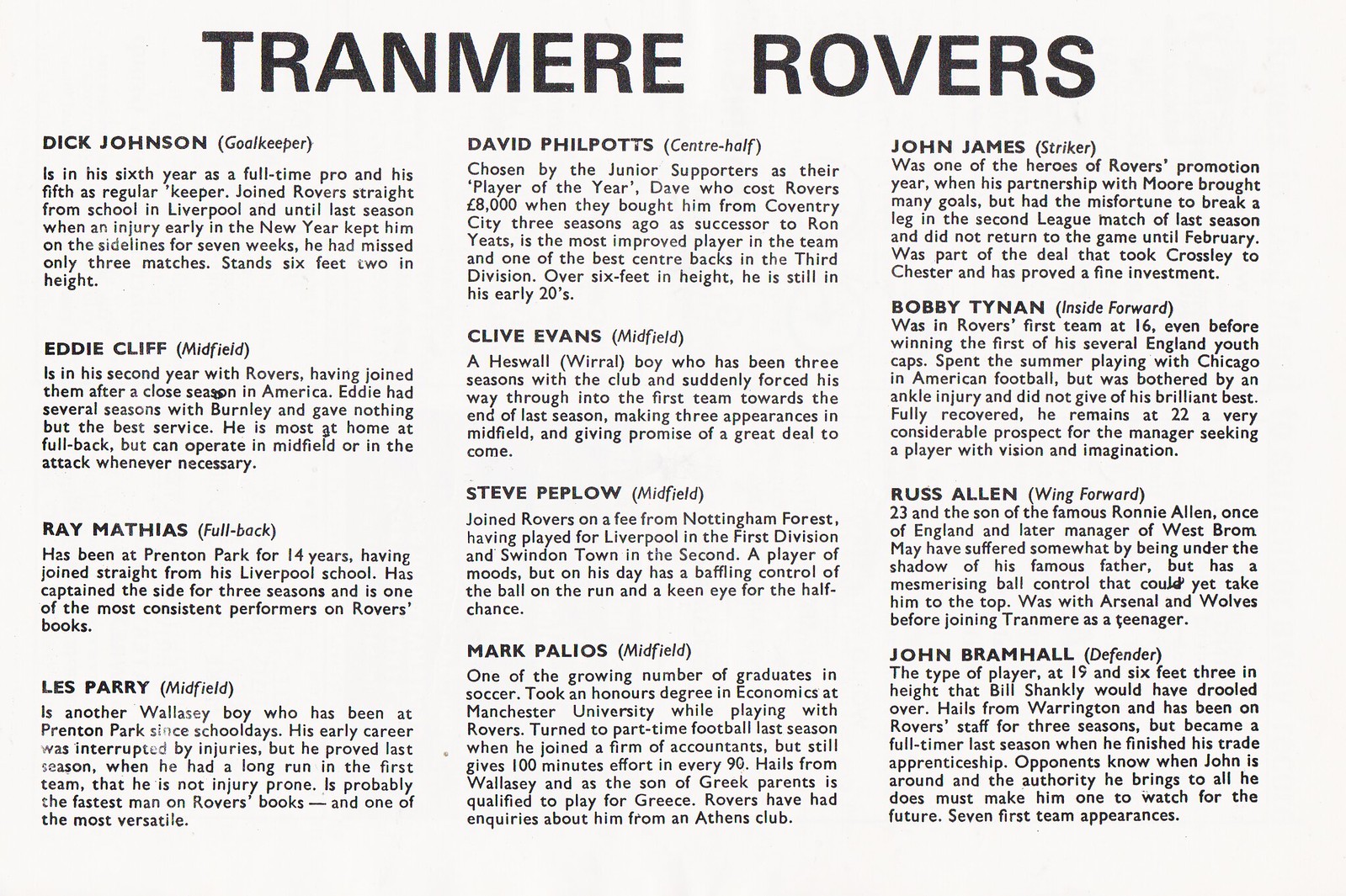The image is a rectangular informational card about the Tranmere Rovers sports team, printed in black text on an off-white background. At the top, large text in all caps reads "TRANMERE ROVERS". The card lists 16 players along with their positions and brief biographical details, arranged in three columns. 

- **Column 1:**
  - **Dick Johnson, Goalkeeper:** In his sixth year as a full-time professional and fifth as a regular keeper, having joined the Rovers straight from school in Liverpool. He stands six feet, two inches tall. Notably, he only missed three matches until last season when an early year injury sidelined him for seven weeks.
  - **Eddie Cliff, Midfield:** In his second year with the Rovers, having joined after a close season in America. Formerly with Burnley, where he provided exemplary service and can also play fullback or in attack.
  - **Ray Mathias, Fullback:** At Penton Park for 14 years, he joined directly from his Liverpool school.
  - **Les Perry, Midfield**

- **Column 2:**
  - **David Philpotts, Center Half**
  - **Clive Evans, Midfield**
  - **Steve Peplow, Midfield**
  - **Mark Pellios, Midfield**

- **Column 3:**
  - **John James, Striker**
  - **Bobby Tynan, Inside Forward**
  - **Russ Allen, Wing Forward**
  - **John Bramhall, Defender**

This detailed roster provides a thorough view of the team, highlighting individual player roles and contributions.